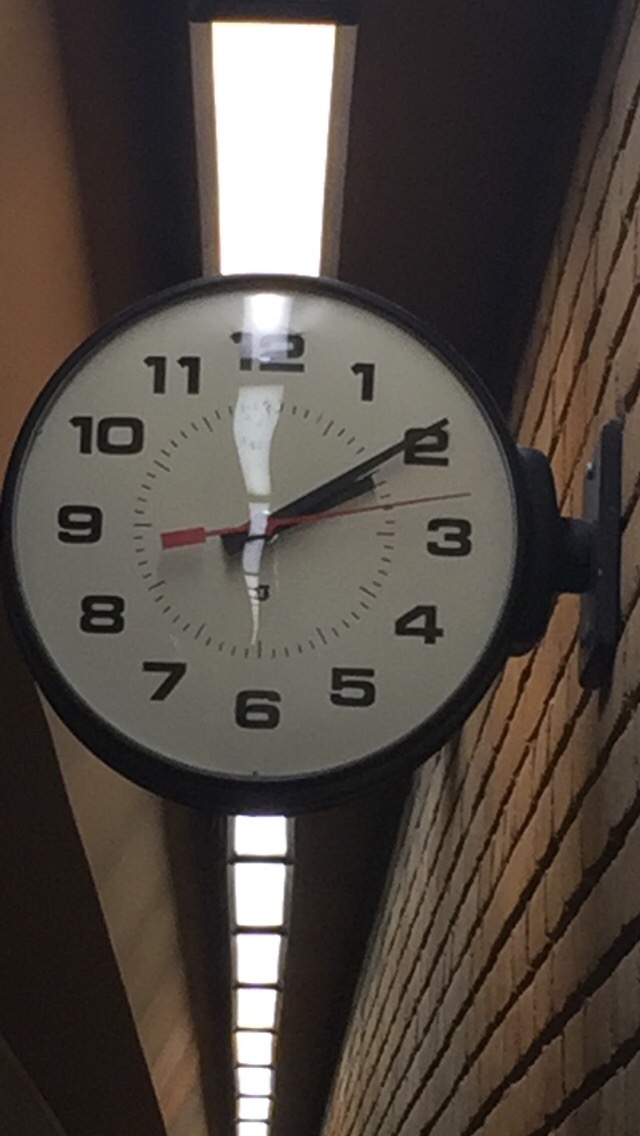This photograph captures a vintage-style wall clock securely mounted on a brick wall to the right. The clock is affixed by a robust black metal bracket, which complements its elegant black metal border. The clock’s face is a pristine white, featuring bold black numerals and hash marks that clearly delineate the hours. Both the hour and minute hands are pointing toward 2, while the slender red second hand is positioned between the 2 and the 3. The scene is subtly illuminated by a row of fluorescent lights running down the hallway, casting a soft glow on the brickwork and creating a timeless, serene ambiance.